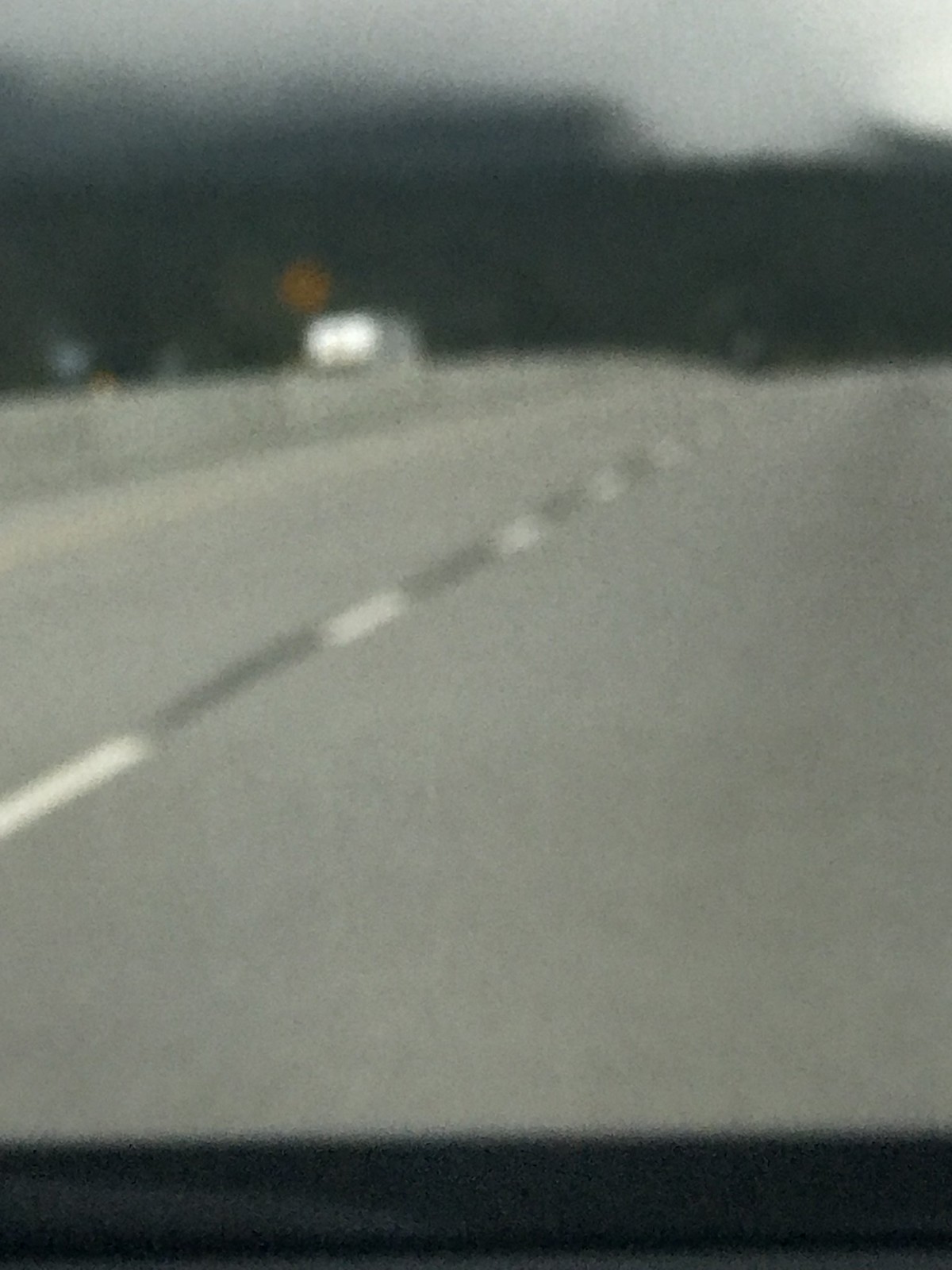This image is very blurry and predominantly dark, making it challenging to discern specific details. The overall composition appears mostly gray. The photo captures a highway scene under a light gray sky. On the horizon, there are indistinct dark gray shapes that likely represent trees, and a more uniform dark gray line, possibly an overpass. In the distance, there appears to be a vehicle on the right side and possibly a white van on the left. Above the white van, there is a small gold circle, and further to the left, a blue circle is visible. The highway itself is a light gray asphalt with a white dotted line marking the middle of the two discernible lanes. At the bottom of the image, there is a black strip that might be part of the vehicle from which the photo was taken.